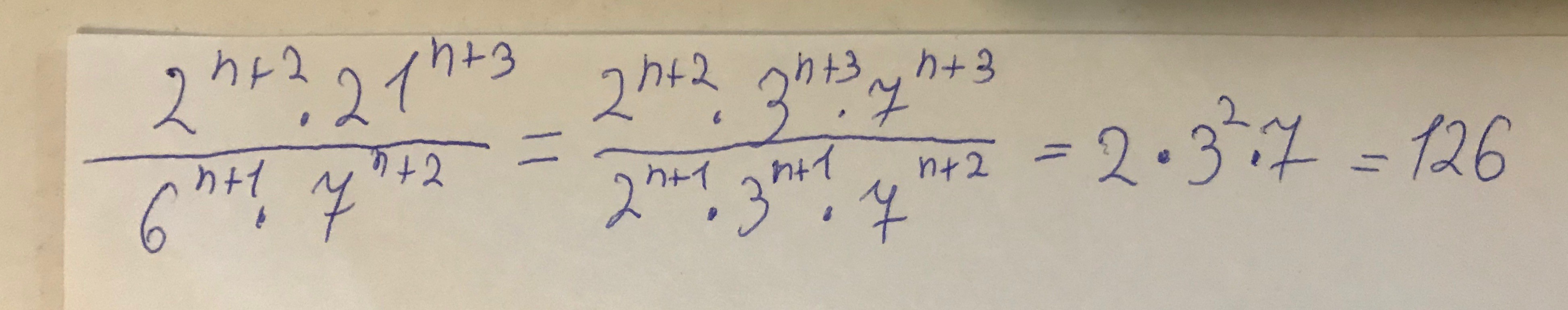This is a horizontal, rectangular photograph capturing a segment of a math equation written on white paper. The paper itself is set against a white background, with a subtle shadow running along its top and side edges, providing a bit of depth to the image. The mathematical notations are penned in blue ballpoint ink. The equation appears complex and somewhat unintelligible, featuring various combinations of numbers and variables. It includes expressions such as \(2H + 2.27\), \(21H + \frac{3}{6H + 1}\), and \(7H + 2 = 2H + 2.3H + 3.7H + \frac{3}{2H + 7.3H + 7} + 7H + 2 = (2.3)^2\). The figure "126" is mentioned, likely as a part of the equation's solution or result.